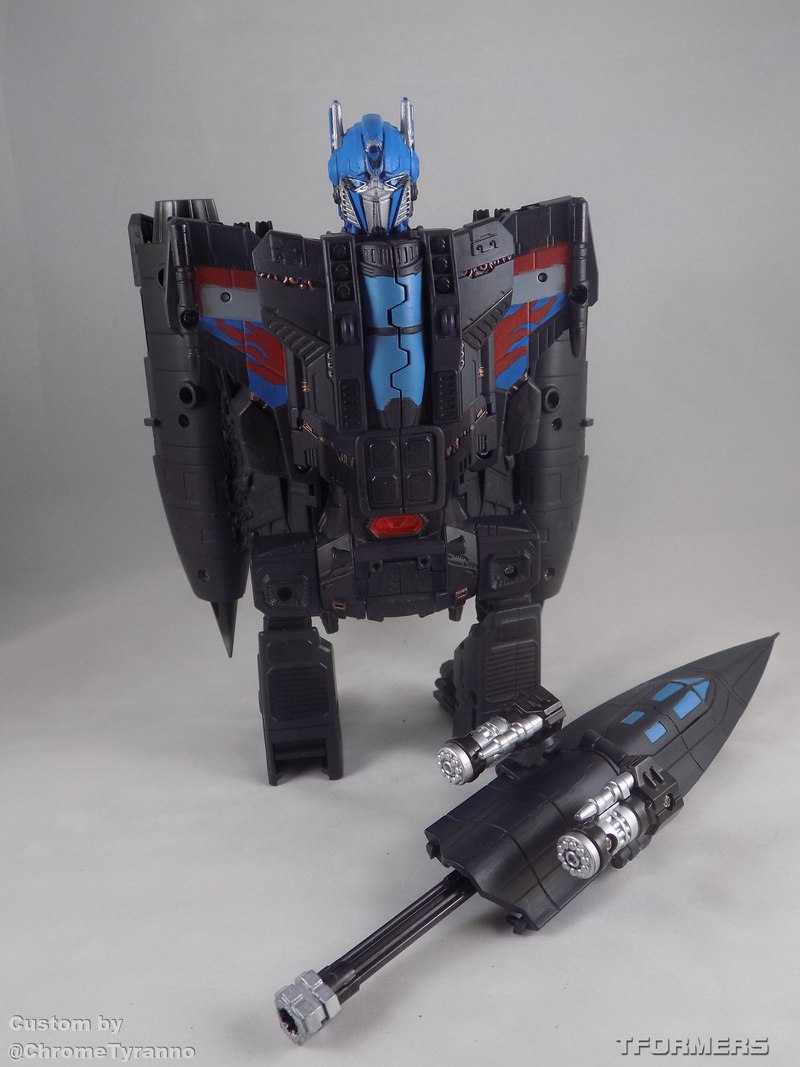In the image, there is a highly detailed transformer toy designed to resemble both a robot and a futuristic vehicle, evocative of those from Star Trek. The toy predominantly features black limbs and a blue torso, with a distinctive blue helmeted head that has silver areas where a face would be, complemented by silver horns on either side of the helmet. The robot's wings, which could also be interpreted as part of a jet's structure, extend outward from where its neck would be. 

In the foreground of the image, there is a secondary piece that appears to be the nose cone of a jet. This piece is black with blue accents, including blue windows and a blue cockpit with a black pointed nose. The attachment suggests it fits onto the primary toy, converting it from a robot back into a complete jet. The wings of the toy appear to function as jet propellers when fully transformed into vehicle mode. 

The toy and its additional components are marked with the text "Custom by Chrome Tyrano" at the bottom left and "Tformers" at the bottom right, giving credit to its custom design. The background of the image is gray, emphasizing the toy's details and colors.